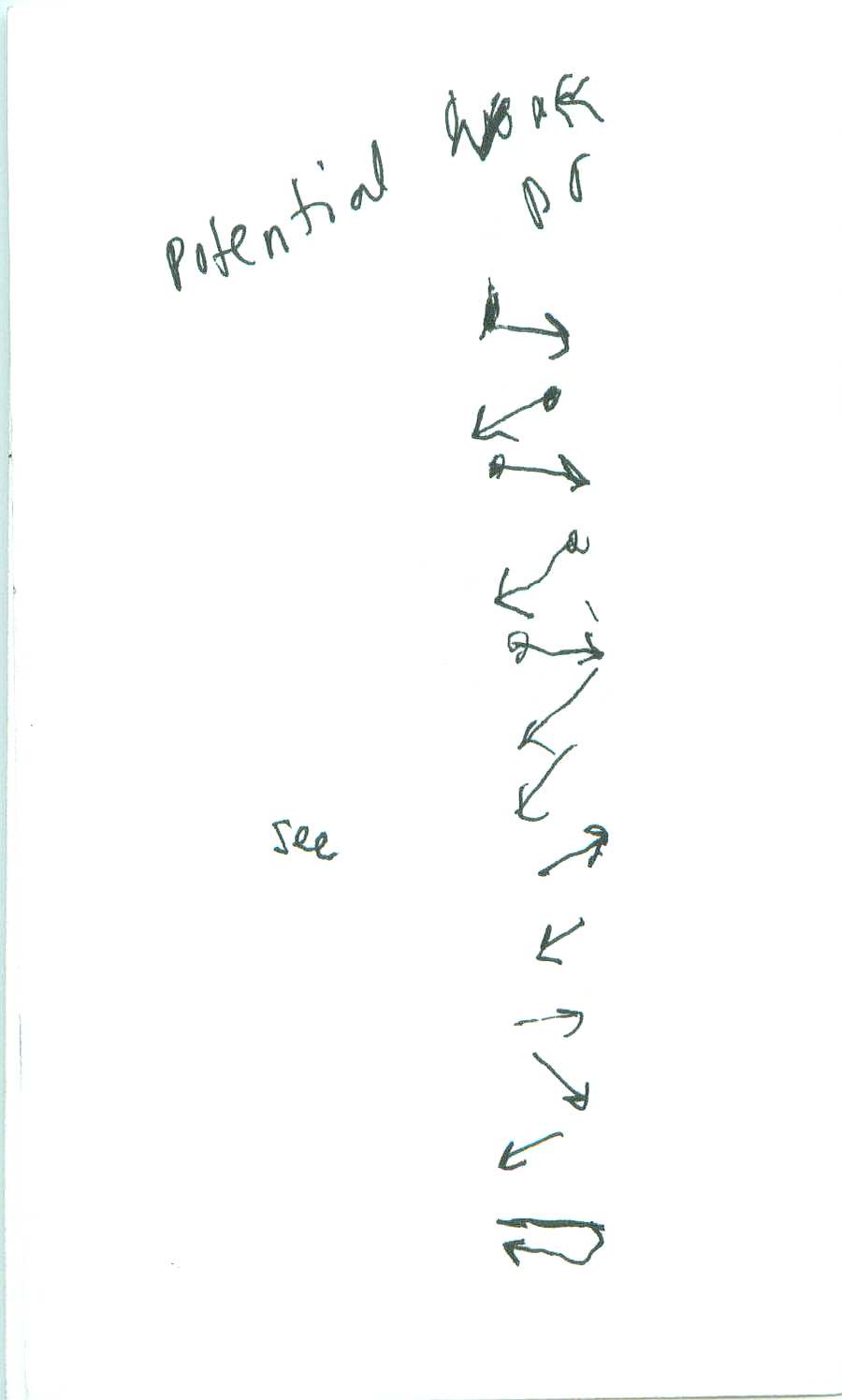The image features a piece of white paper filled with black ink or marker writing arranged vertically. At the top of the page, the word "potential" is written, followed by a word that appears to be "work," although it is spelled inaccurately as "W-O-A-K." Below that, the letters "P" and "D" are faintly visible, though their exact identification is uncertain. The majority of the page is filled with a series of alternating directional arrows. From top to bottom, these arrows point right, left, right, left, right, left, left, right, left, right, and left. At the bottom part of the page, a horizontal line stretches from left to right, followed by a continuation of the arrow pattern that curves in a horseshoe shape, turning back to the left. To the right of this vertical sequence, the word "C," spelled out as "S-E-E," is written. The document has no visible background or context beyond the black words and arrows on the white paper, creating a stark, minimalist presentation.